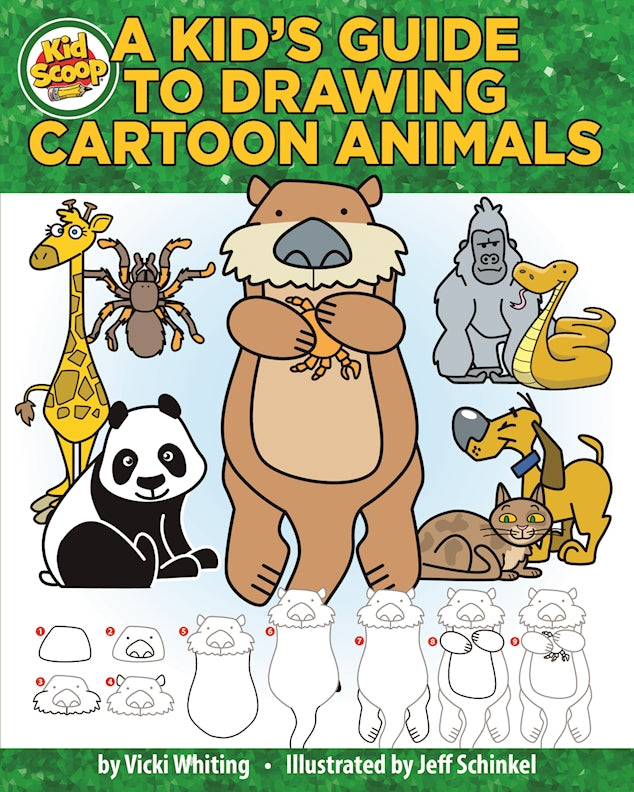This image is the cover of a book titled "A Kid's Guide to Drawing Cartoon Animals," prominently displayed in all caps, yellow bubble letters outlined in black, set against a green, tree-like textured background. At the top left, partially overlapping the green background, there's a white circle with "Kid Scoop" written in orange and set against a red background. The focal point of the cover is a collection of colorful, hand-drawn animals including a giraffe, a panda, a dog, a cat, a gorilla, a snake, a spider, and an otter holding a crab, all set against a very pale blue or white background. At the bottom of the cover, a green strip mirrors the top background and contains the text "By Vicki Whiting, Illustrated by Jeff Schinkel" in white letters. Just above this text, there's a detailed step-by-step drawing guide for creating the otter, starting from simple shapes and gradually adding details, accompanied by red numbered circles guiding the process.